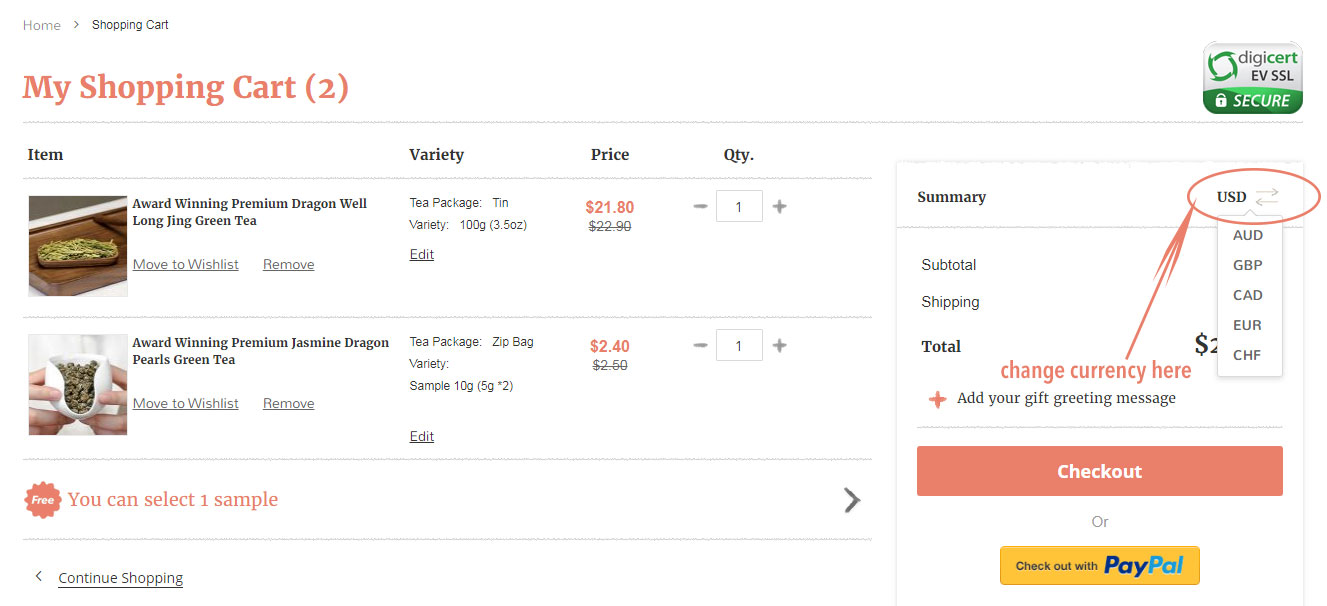A screenshot of a shopping website is displayed. In the top left corner, the navigation options "Home" is followed by a right-facing arrow and then "Shopping Cart," all in gray text. Below this, the section is titled "My Shopping Cart" with the number "(2)" in red, indicating two items.

The first item listed begins with the word "Item" in gray on the far left. Directly below this is the product name "Award-Winning Premium Dragon Well, Longjing Green Tea," accompanied by a thumbnail image that is too small to discern specific details. Beneath the product name, there are options to "Move to Wish List" or "Remove" the item. Moving to the right, under the heading "Variety," the details specify "Tea Package, Tin Variety, 100g (3.5 ounces)," with an option to "Edit" immediately below. To the right under the heading "Price," the cost is displayed as "$21.80" in red text. Further right under "Quantity (QTY)," a box features a "-" sign to the left, a "+" sign to the right, and the number "1" in between.

The second item in the cart is listed next. In bold black letters, the product name is "Award-Winning Premium Jasmine Dragon Pearls Green Tea." Below the name, the options "Move to Wish List" and "Remove" are available. Under the "Variety" heading to the right, the product is described as "Tea Package, Zip Bag Variety, 10g (0.35 ounces)," with an "Edit" option below. Continuing right under "Price," the cost is shown as "$2.40" in red text. Lastly, under "Quantity (QTY)," a box shows the number "1" with a "-" sign to the left and a "+" sign to the right.